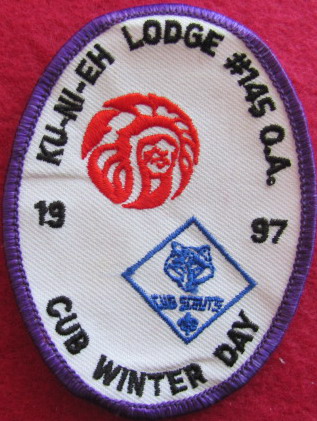This is a detailed photograph of an oval-shaped, hand-sewn patch. The patch features a thin purple border stitched around its perimeter, which encircles a white background. Prominently situated across the top in a black arching text is "KU-NI-EH Lodge No. 1450.A." Below this, in the center, is the year "1997" flanked by the number "19" on the left and "97" on the right. The bottom arch reads "Cub Winter Day." 

Dominating the center of the patch is a red logo depicting a Native American chief adorned in a full headdress. Additionally, there's a blue diamond-shaped emblem with the words "Cub Scouts" and the image of a wolf. The patch is laid out on a soft, reddish-magenta felt material, which adds a warm, vibrant background to the detailed patchwork.